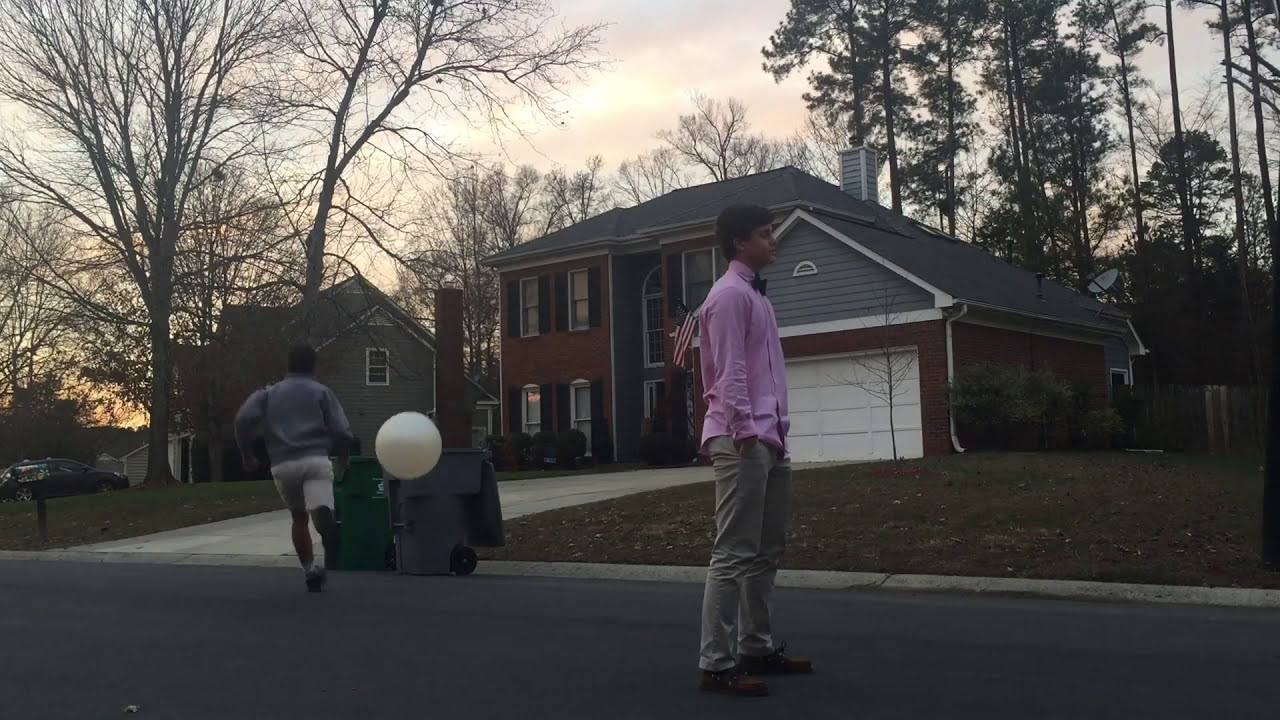In this early evening outdoor photograph, the scene unfolds in a quiet residential neighborhood under the warm hues of a sunset sky. Prominently, a young man, approximately 20 years old, stands steadfast in the middle of an asphalt-paved street. His dark hair is neatly styled, and he wears a pink button-down shirt, slightly untucked, paired with khaki dress pants and light brown dress shoes. A stylish black bow tie accentuates his outfit. His right side is mostly facing the camera, with his hands casually tucked into his pants pockets, and he gazes towards the right center of the image.

To the far left, another young man, donned in a black or gray sweatshirt with khaki shorts and black shoes, is caught in motion as he chases a ball towards a driveway. His back is turned to the camera, adding a sense of dynamic movement to the scene.

In the background stands a large, two-story red brick house with gray siding and a gray-tiled roof. Near the garage of this house flutters an American flag on a pole. Beside the driveway, there are two large trash cans, one green and one gray with wheels, positioned on the street.

Behind the houses, tree branches, both barren and leafy, stretch out against the twilight sky. The sunset bathes the clouds in a serene orange glow, casting long shadows and adding depth to the image. This meticulously captured moment encapsulates the tranquility and subtle activity of suburban life at dusk.